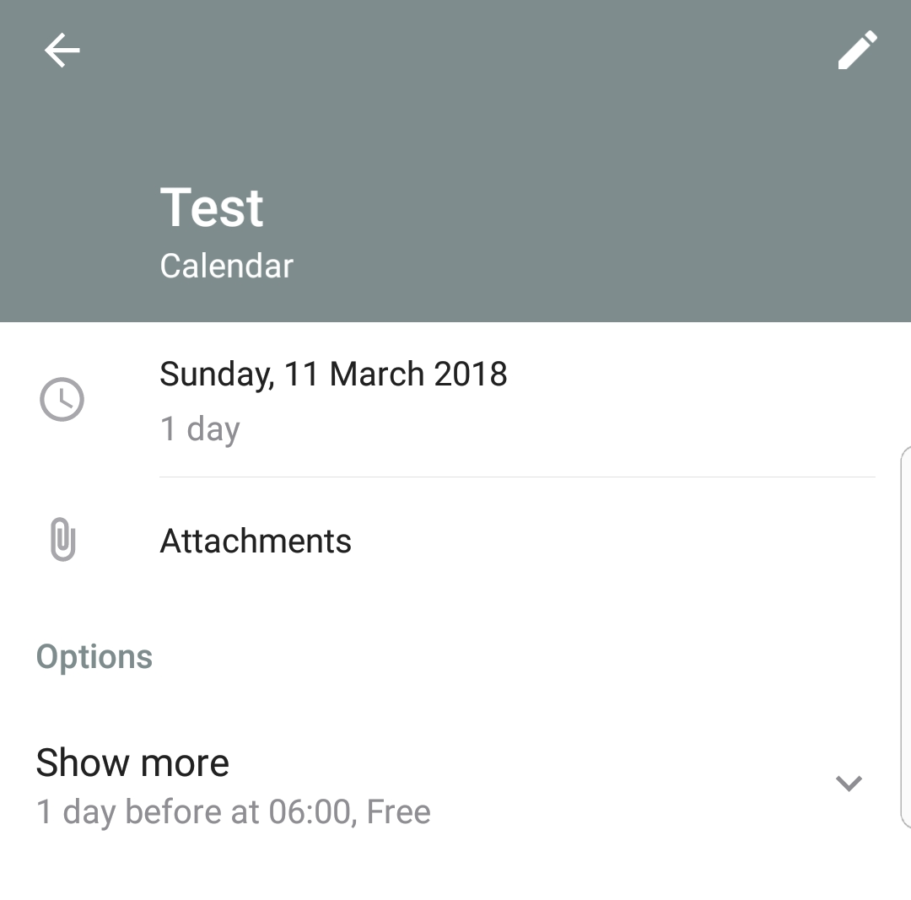This image is a detailed screenshot of a calendar application interface, divided into several distinct sections. 

**Upper Section**:
- The topmost portion features a horizontal gray background spanning from the upper left to the upper right corner. 
    - In the upper left corner, there is a back arrow icon.
    - In the upper right corner, there is a pen icon symbolizing an edit function.
- Between these icons, the text reads "Test Calendar" indicating the title of the calendar event.

**Main Content Area**:
- Below the gray header, the main content begins with a large white section.
    - On the left side, there is a clock icon, indicating the scheduled day and time of the event.
    - Next to the clock icon, the date "Sunday, 11th March 2018" is written in black text.
    - Beneath the date, in a smaller gray font (which is harder to read due to contrast), it specifies "one day."
- A faint gray line separates the date section from the subsequent information.

**Additional Information**:
- Below the separator, the left side features a paperclip icon, denoting attachments related to the calendar event.
    - Adjacent to this, the word "Attachments" is prominently displayed.
- The next row mentions "Options," likely related to additional settings for the event.
    - Underneath, the phrase "Show More" is written in black text, possibly indicating expandable details.
- Further down, the text "One day before at 6:00 PM, Free" appears, specifying the status of availability a day prior to the event.

**Summary**:
- The bottom of the screenshot reiterates the availability status: "One day before at 6:00 PM, Free," confirming no engagements at that time.

The interface is cleanly divided into a gray header for quick navigation and an expansive white section for detailed event information.